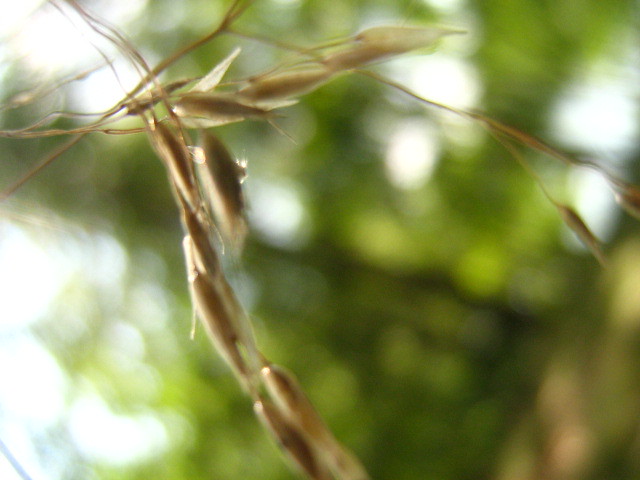In this full-color outdoor photograph taken on a sunny day, the primary focus is a close-up of plant stalks, likely wheat, barley, or similar grains, adorned with seeds. These tan, elongated seeds form the central subject of the image, occupying the left portion and extending slightly to the right with a small branch. The background is richly blurred, creating a soft, dreamy effect that features varying shades of green likely from leaves or other foliage, interspersed with circles of white sunlight and patches of bluish-white that suggest a bright sky peeking through. The scene conveys a serene, natural setting bathed in light.